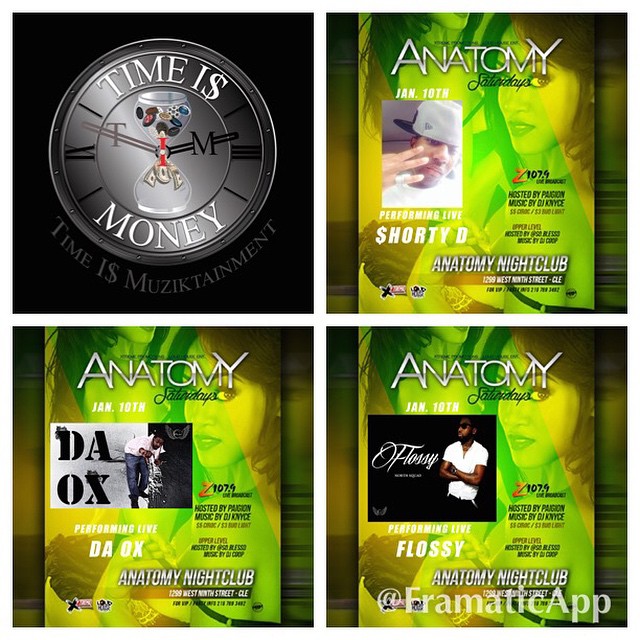The image is a composite of four quadrants, each contributing to a promotional ad for the Anatomy Nightclub. In the top-left quadrant, a dark silver clock with an hourglass at its center is depicted, accompanied by the phrases "Time is Money" (with the 'S' replaced by a dollar sign) and "Time is Music Tainment." This visually striking element emphasizes the value of time and the musical entertainment on offer. The top-right quadrant features a green-tinted poster advertising "Anatomy Saturdays" at Anatomy Nightclub, located at 1259 West 9th Street in Sealy, and highlights a performance on January 10th hosted by radio station Z107.9. The bottom two quadrants showcase variant posters of the same event, each spotlighting one of the three performers: Shorty D, Da Ox, and Flossie, all set to perform live on January 10th. Each quadrant collectively emphasizes the theme of musical entertainment and hypes up the upcoming event at the nightclub.